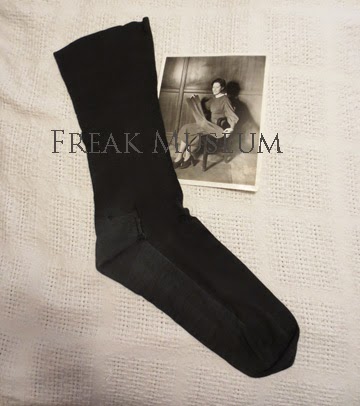The image is a detailed, indoor photograph showcasing a black sock laid out on a flat, white blanket. Adjacent to the sock, on the right, is an old black-and-white photograph of a woman seated in a chair. The woman, dressed in high-heeled shoes and a light-colored dress, is holding the same large black sock, which is notably bigger than her torso, implying its oversized nature. The background of the photograph features a wood-paneled wall and a tiled floor, suggesting an early 20th-century setting. Superimposed over this composite image is the gray, pixelated text "Freak Museum," which partially blends with the sepia tones of the black-and-white photograph, making some of the text difficult to discern.